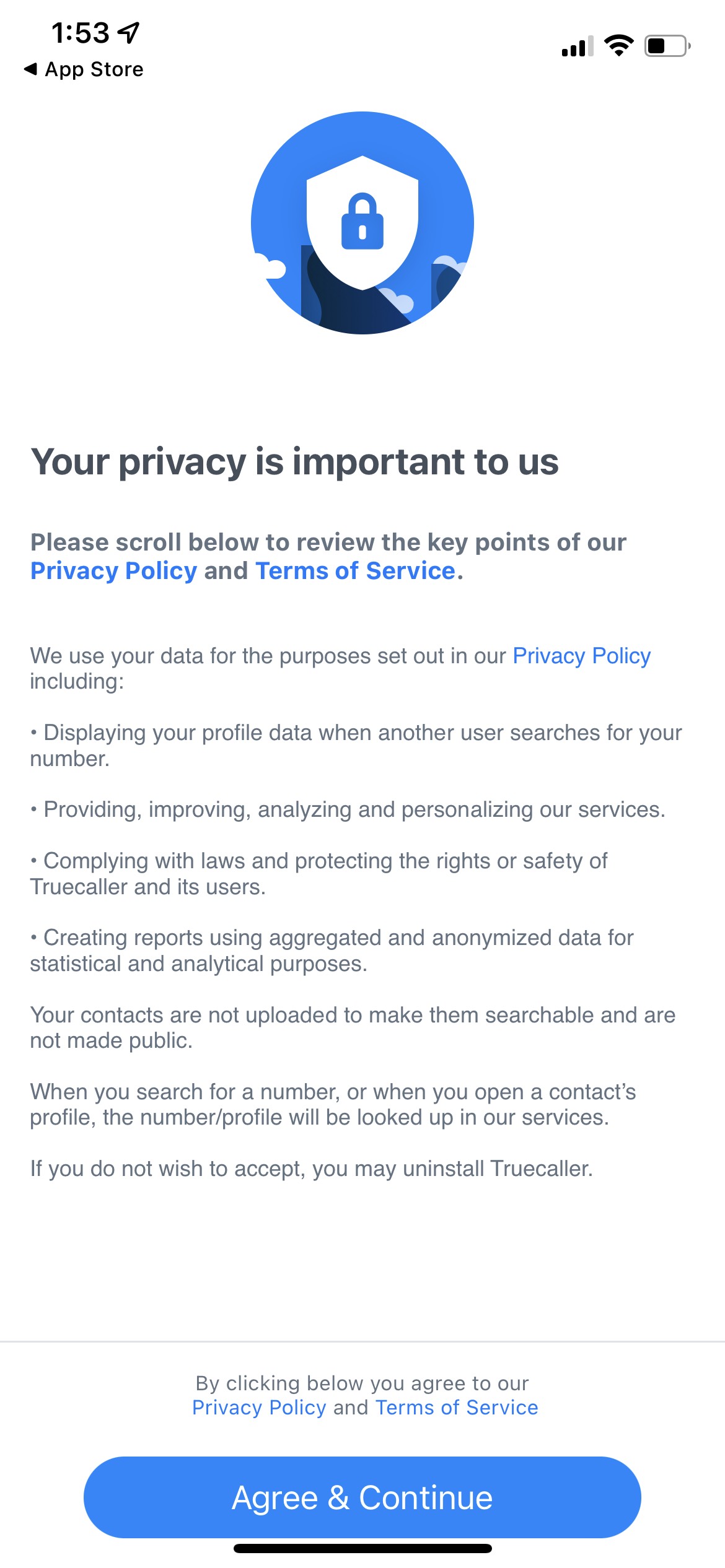At the top of the image, the number "153" is displayed prominently, with the "App Store" label positioned directly below it. The top-right corner features a status bar showing a Wi-Fi symbol with three to four bars, and a battery icon indicating roughly one-third charge remaining.

The central portion of the image showcases a serene scene with a blue sky and a few scattered clouds. Dominating this setting is an icon of a shield with a blue lock inside it, suggesting security and protection.

Below this icon, in bold black text, are the words: "Your privacy is important to us." Underneath, in regular text, the message reads: "Please scroll below to review the key points of our privacy policy and terms of service." This is followed by a blank line for emphasis.

Continuing, more details in regular text state: "We use your data for the purposes set out in our privacy policy including:" a list follows:

* Displaying your profile data when another user searches for your number.
* Providing, improving, analyzing, and personalizing our services.
* Complying with laws and protecting the rights or safety of Truecaller and its users.
* Creating reports using aggregated and anonymized data for statistical and analytical purposes.

The message concludes with a prompt: "Please scroll below to review the key points of our privacy policy and terms of service."